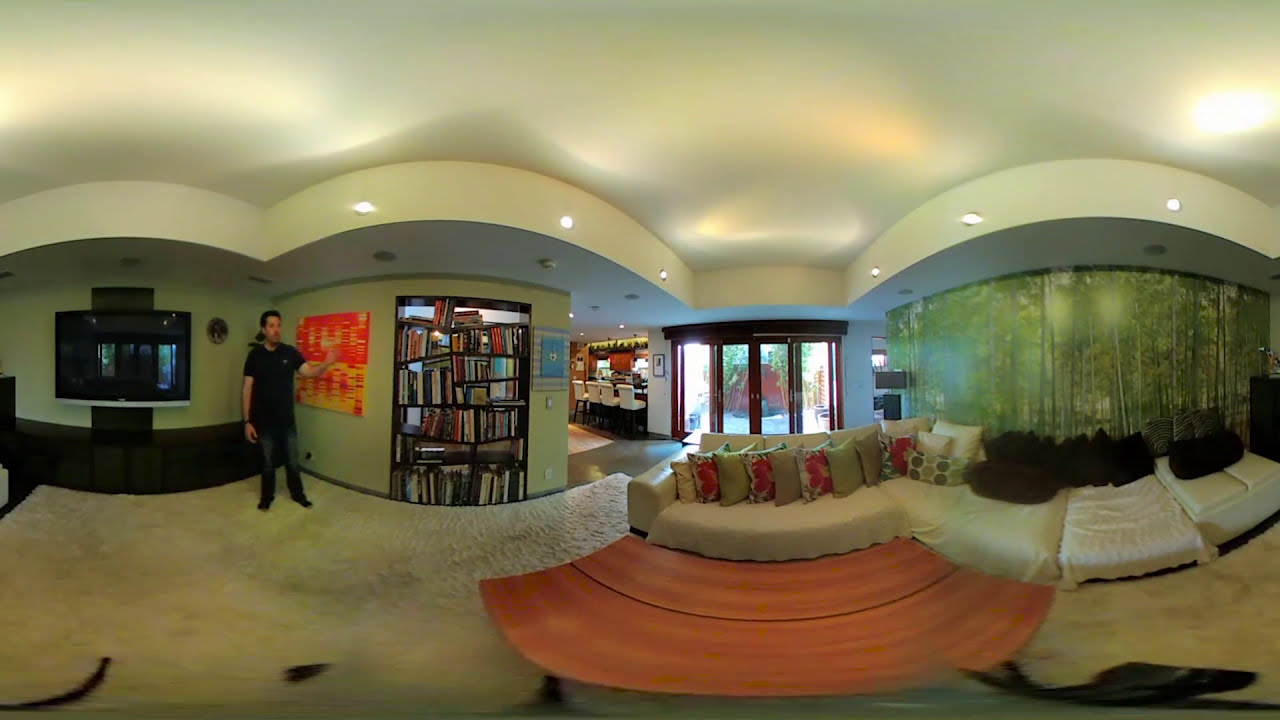The image depicts a horizontally aligned rectangular photograph of a spacious, tastefully decorated living room with clean, gently curved white walls and a ceiling illuminated by spotlights, lending it a grayish hue. Central to the room is a set of glass doors leading outside, flanked by a wallpaper mural of a forest. Three distinct curved wall sections provide a unique architectural interest, with one on the far left, another to its immediate right, and a third on the right side of the image. A large sectional sofa occupies the middle of the room, adorned with an array of green, pink, and floral-patterned throw pillows, and is extended by a footrest area with dark pillows. 

In front of the sofa, set against an ivory or beige shaggy carpet, lies a curved wooden coffee table. The foreground includes a slightly blurred curved wooden piece, possibly an end table. Additional elements include a brown coffee table and a bar area with white stools to the left of the glass doors. A man stands between the first two curved wall sections on the left, dressed in jeans and a short-sleeve black shirt, with short brown hair. He is gesturing as if explaining something, potentially towards the couch area where the sofa and table are situated. On the left side of the image, a bookshelf and a wall-mounted television are visible, completing the inviting scene.